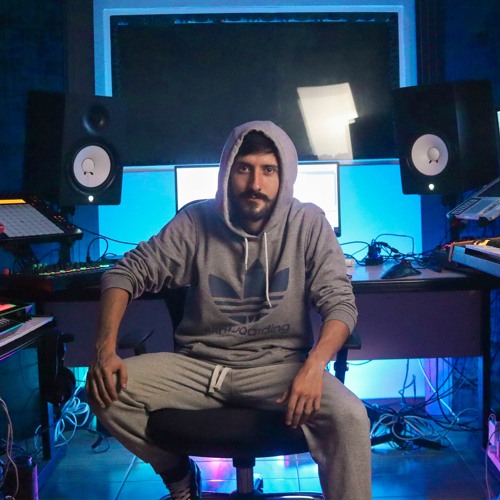A man is seated on a stool, dressed in a gray hoodie adorned with a blue flower and two gray drawstrings, paired with gray sweatpants featuring two white drawstrings. Behind him, a desk supports a computer setup flanked by two large black speakers, each with a prominent white circle in the center. The backdrop reveals a blue-lit screen, possibly a projection board or another large monitor, casting a vivid glow. The floor is illuminated in blue light, with numerous cables scattered on either side. To the left, an additional screen displays grid lines, while to the right, various music production equipment is visible. The man's right foot is clad in a tennis shoe.